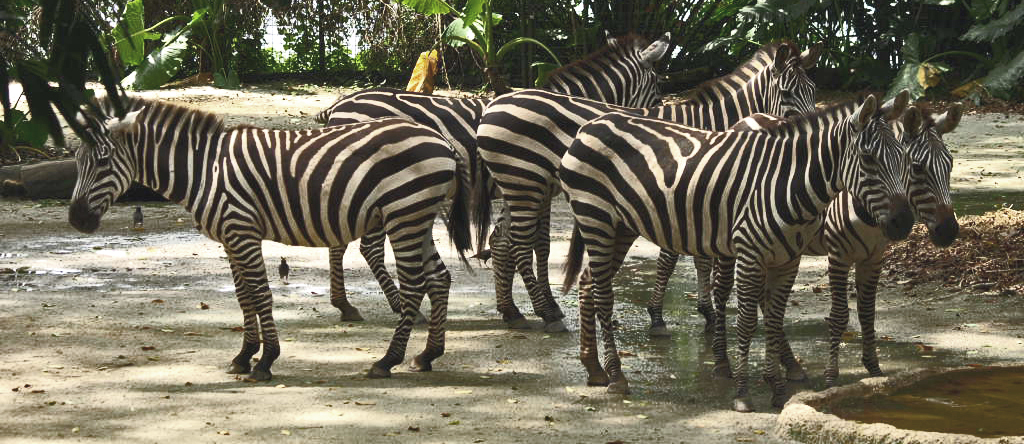The image captures a small herd of five zebras standing close together in a zoo enclosure. The zebras, known for their black-and-white stripes and black tails with tufted ends, are positioned on a flat, light gray, rocky ground with packed beige soil. Most of the zebras are facing to the right, while one zebra is facing to the left, creating a circular arrangement with their bodies. To the right side of the foreground, there is a man-made watering hole or trough with dark brown water, bordered by cement or plaster. Additionally, the ground near the zebras holds two Indian myna birds. The enclosure is outlined with a barely visible thin wire fence on the left, suggesting its artificial setting. Dense green foliage, possibly strelitzias or banana plants, is present in the background, contributing to a lush, tropical ambiance.